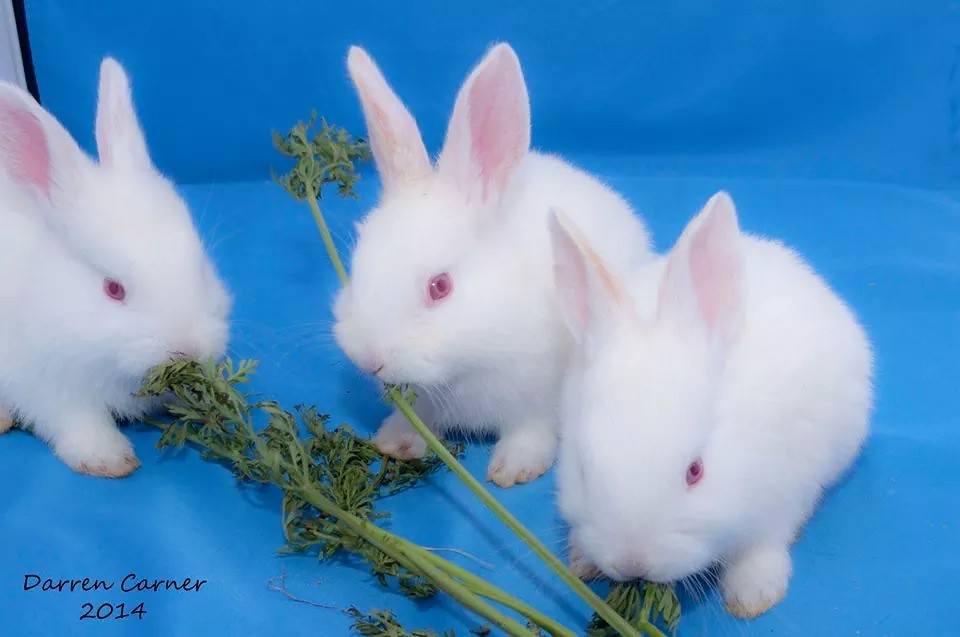A photograph captures three very small, fluffy baby rabbits with pure white fur, suggesting they might be albino, as indicated by their light pink to red eyes and pinkish inner ears and paws. They are all nibbling on a piece of greenery with long, skinny stems and very small leaves, which might be the tops of carrots. The leftmost rabbit is partially cut off by the image and faces inward, the middle one is perked up, and the rightmost one looks downward towards the bottom middle of the photograph. All three are sitting on a bright blue material that extends from the bottom of the image to the background behind them. In the bottom left corner, the name "Darren Karner 2014" is written in black font, identifying the photographer and date.